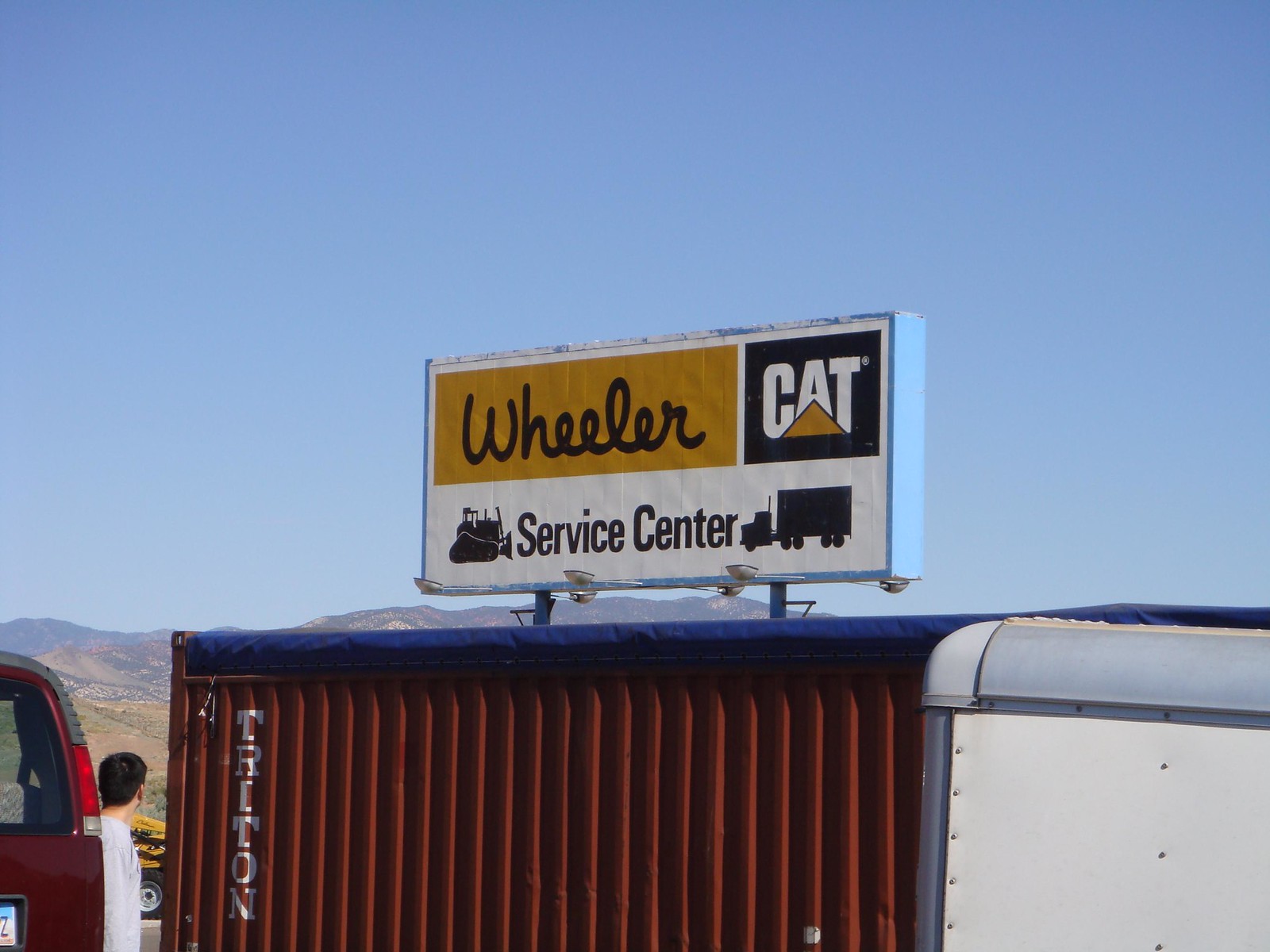This photograph captures an outdoor scene set against a backdrop of clear, light blue skies and brown, rugged hills, suggesting a location in the southwestern United States, possibly Southern California, Arizona, or Nevada. In the foreground, a large red storage container with pleats and a blue roof is prominently featured. The container is adorned with silver capital letters spelling out "Triton" vertically near its left edge.

Rising behind this container is a billboard sign for Wheeler Service Center. The sign features a golden-yellow background with "Wheeler" written in black script on the left and a black square with "CAT" in white letters on the right, featuring a pyramid within the "A." Below this, "Service Center" is written, flanked by a black depiction of a tractor on the left and a semi-truck on the right.

To the right of the red container's front corner, a small portion of a white trailer with gray trimming is visible, suggesting additional storage or utility equipment. In the lower-left corner, the bronze tailgate of a vehicle, likely a minivan, is seen with a sliver of a license plate and reflector lights alongside the rear window.

Between the red storage container and the van, a young man wearing a gray shirt stands, gazing out towards the distant hills. A tiny glimpse of bright yellow construction equipment, likely CAT-branded land-moving machinery, peeks out near the man. The entire scene evokes a sense of industrial activity against a stark, expansive desert landscape.